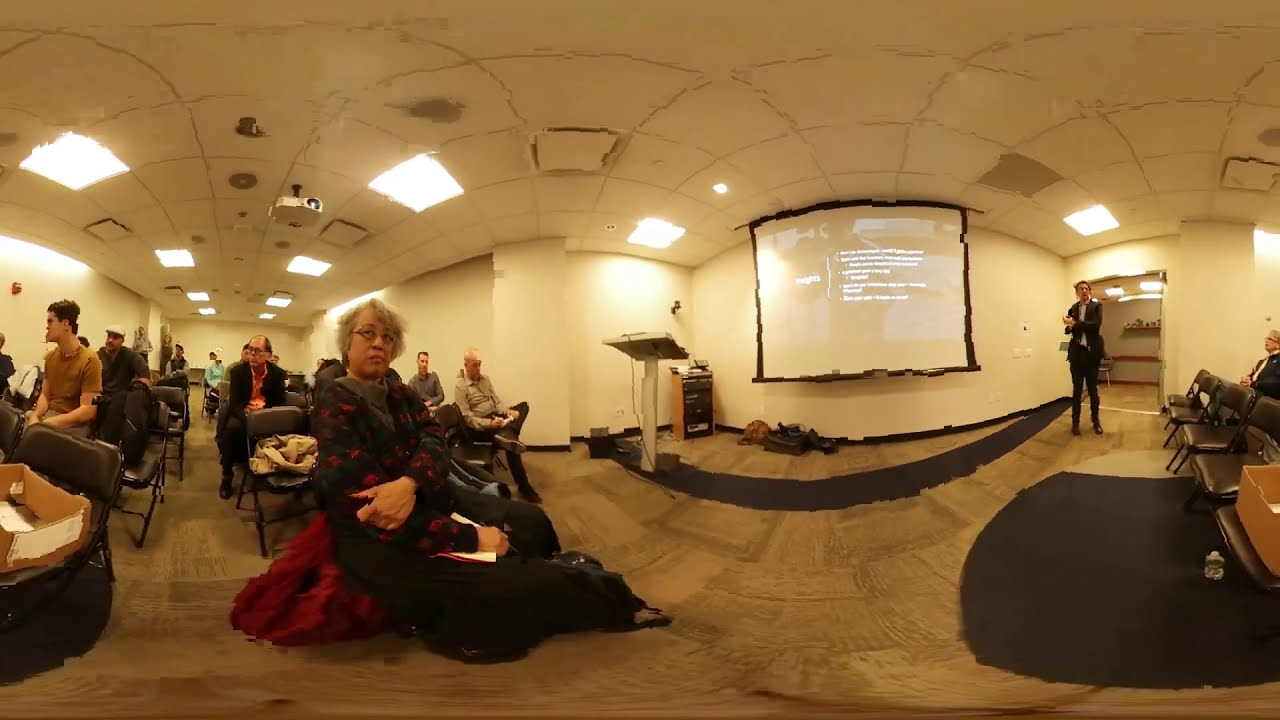This image depicts the interior of a conference room or possibly a church, characterized by a light tan cast that permeates the entire space, including the ceiling, walls, and the darker tan floor. Centrally positioned is a small, dark tan stage just to the right of center, which includes a light tan podium. Above and behind the stage, hanging from the ceiling, is a large screen trimmed in black, displaying a PowerPoint slide. The slide features the word "Hughes" along with several bullet points, shown in clear, bold, white font against a beige background. In front of the screen, a man dressed in a black suit jacket, pants, and shirt stands to the right and appears to be clapping his hands and speaking, potentially addressing the audience. The room is filled with rows of dark grayish-black chairs in which people are seated, attentively watching the presentation. The bright ceiling lights illuminate the room, adding to the slightly distorted, circular angle of the image, which gives the appearance of being stretched.